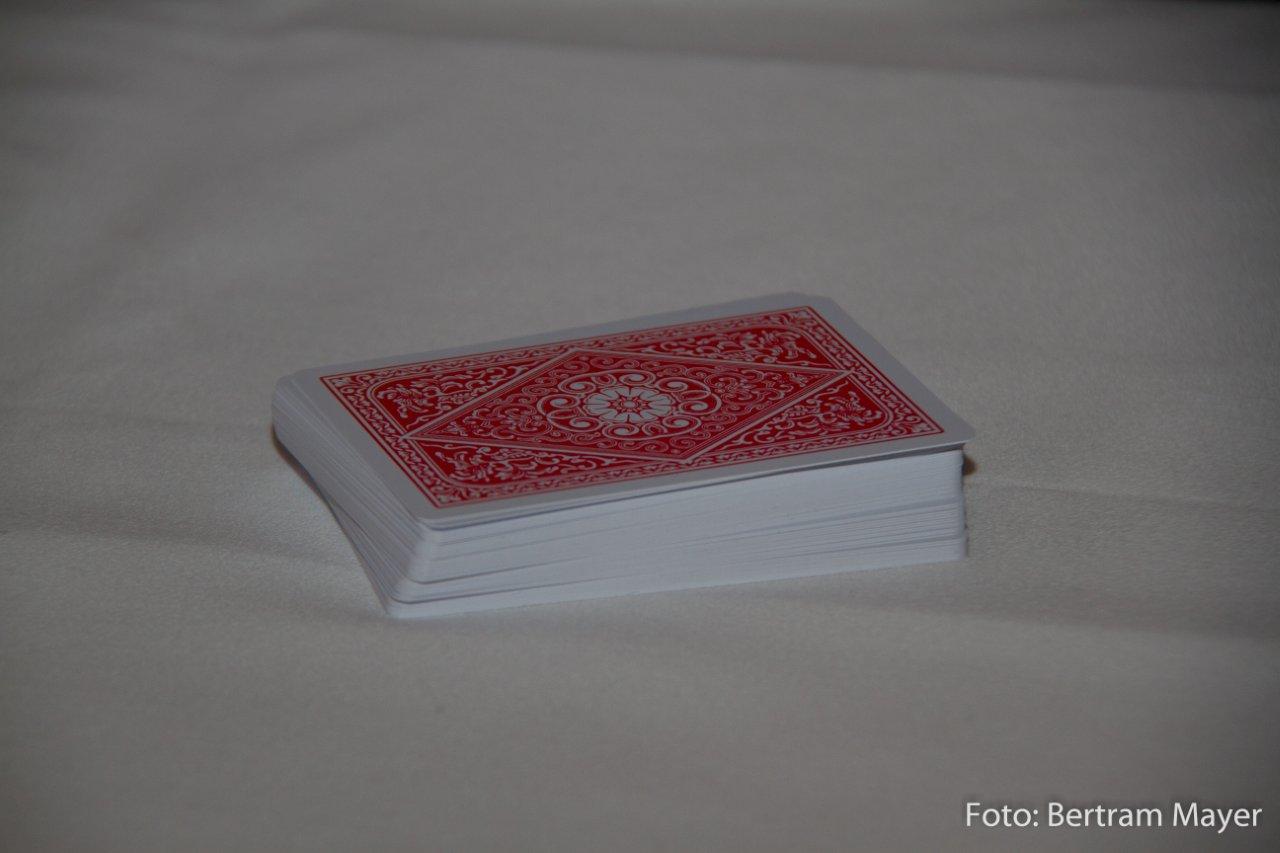In the image, a deck of cards is elegantly positioned on a white cloth that spans the entire picture. The cloth stretches from the top left corner to the bottom right in a diagonal fashion. In the upper left corner, approximately an inch from the top, there is a noticeable fold in the cloth. The top right corner of the image features a darker, shadowy area that also descends about an inch before the shadow veers off to the side, creating a striking contrast against the white background. Midway through the cloth, a subtle crease about an inch wide can be observed, stretching diagonally from left to right, with a slightly darker hue than the rest of the fabric.

Atop this crease lies the deck of cards, oriented horizontally with one side facing the left and the top side facing the right. The cards are slightly turned in the distance, creating a gentle, almost imperceptible fan. Each card boasts a white border with a vibrant red square adorned with intricate designs. Within this red square, a red diamond, outlined in white with additional red embellishments inside, captures attention. In the bottom right corner of the image, a caption reads "FOTO.. Bertram Mayer," indicating the artist behind this captivating composition.